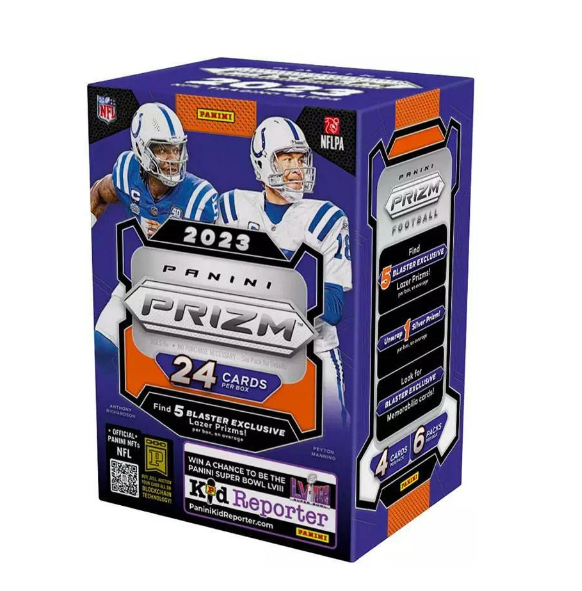The product is a box of 2023 Panini PRIZM NFL Football Trading Cards, which contains 24 cards. This rectangular box features a blue background and prominently displays two football players in their respective team uniforms. On the left, one player wears a light blue jersey with white stripes and a white helmet, while on the right, the other player dons a white jersey, marked with the number 18, and a white helmet with an upside-down horseshoe bordered by a blue stripe. At the top left corner, the box features the NFL logo, and to its right, the NFLPA logo. A black tab near the top indicates the year 2023, followed by the product name "Panini PRIZM" and the content "24 cards." The packaging also mentions the inclusion of five blaster exclusive laser prisms and has a QR code for additional digital content. There is a reference to a "Kid Reporter" contest related to the Super Bowl, adding to the collectible nature of the product.